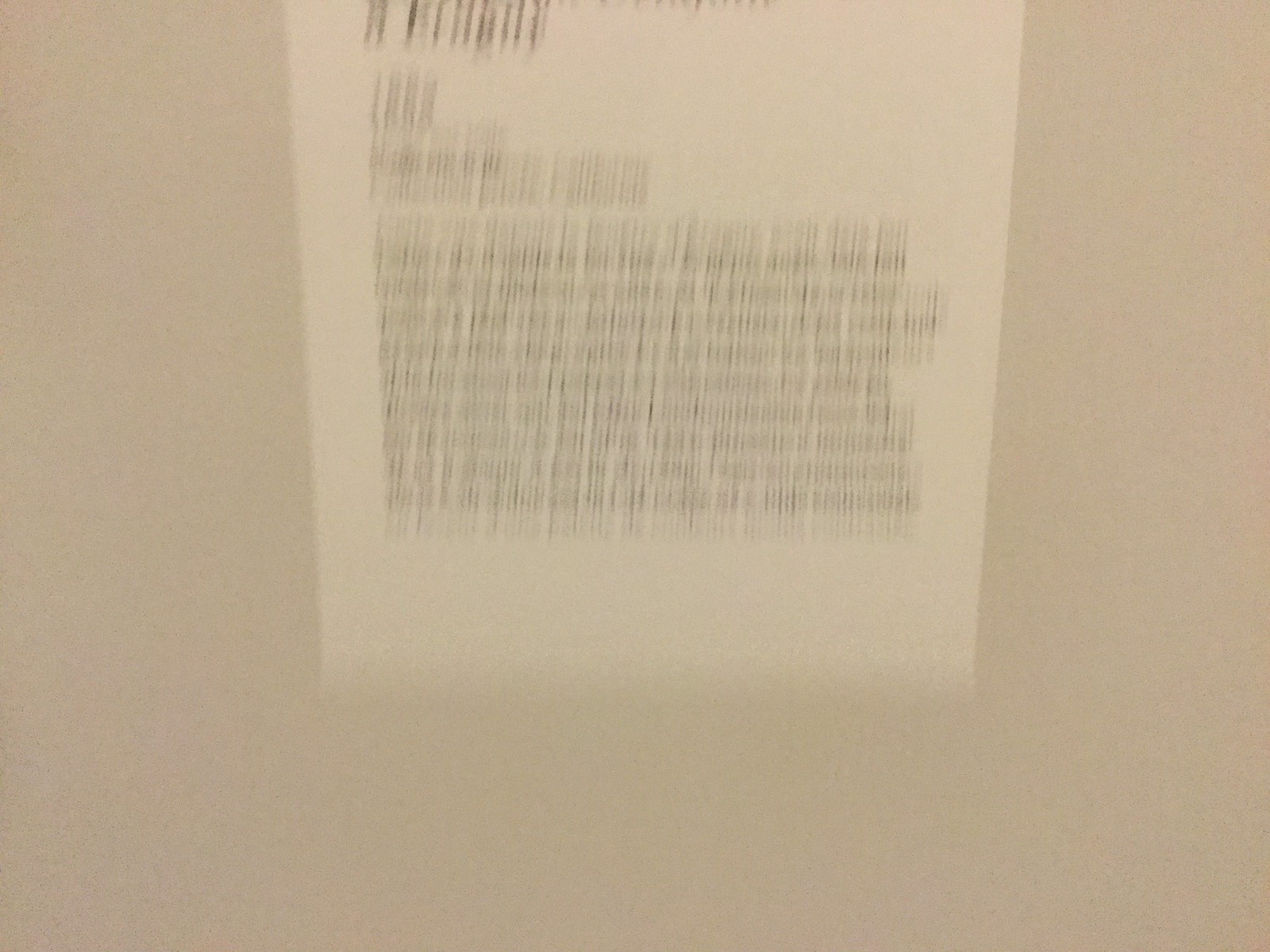The image features an off-white or very pale gray background, possibly a wall or a flat surface. At the center is a white piece of paper resembling the bottom section of a receipt or a notice, somewhat off-kilter and not perfectly aligned within the frame. This paper has blurry black text suggesting a paragraph and a couple of smaller lines, yet the wording is illegible due to significant motion blur, possibly caused by the camera movement during capture. The overall image lacks distinct detail, with a ghostly or grainy quality to both the background and the paper, making it impossible to discern any specific information from the text.